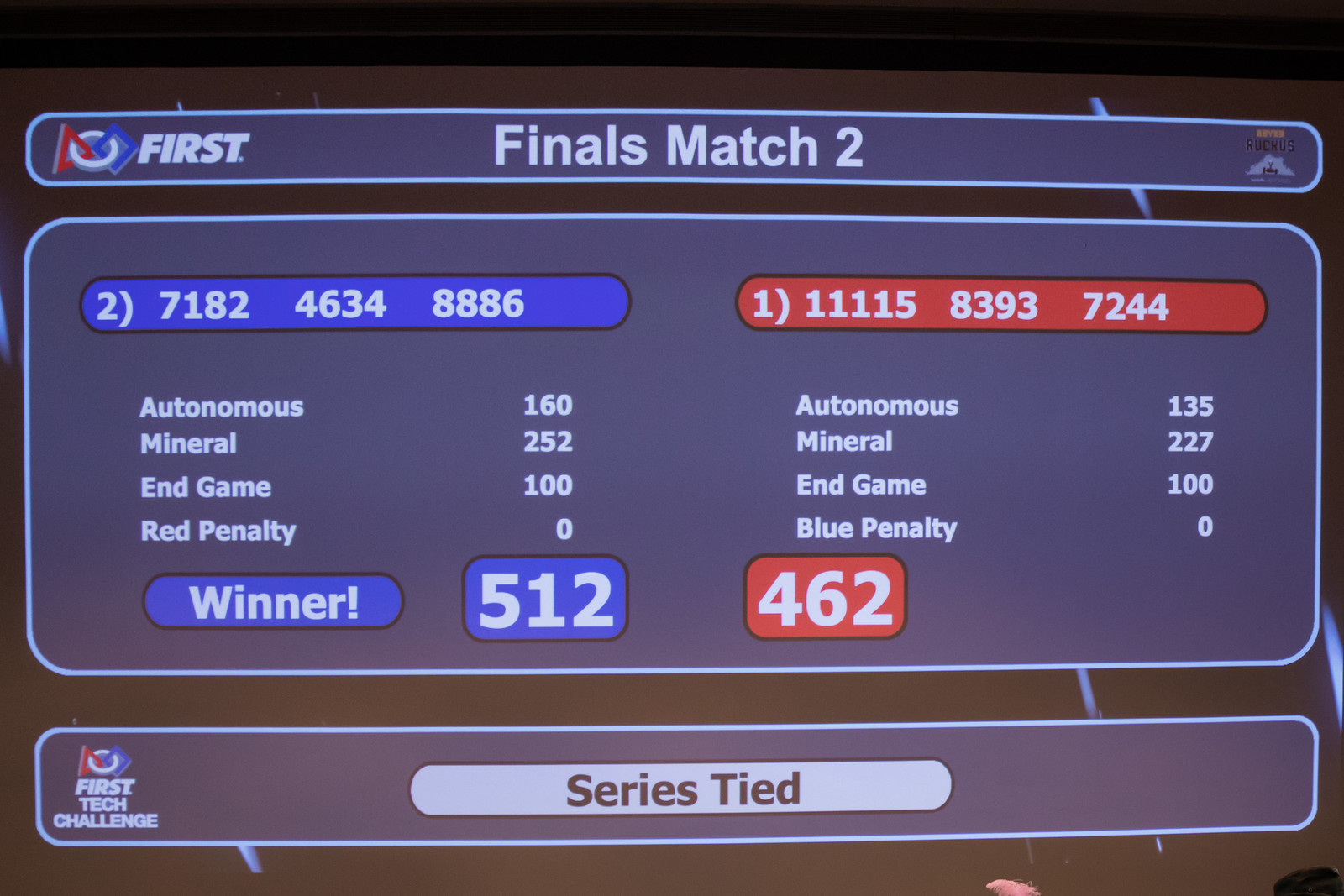The image is a photograph of an older television screen displaying a digital scoreboard in landscape orientation. The scoreboard is divided into three horizontal sections, each wider than tall. The top section, a narrow black band, features the white text "First Finals Match 2" centered within it. Below, the main body of the scoreboard has a brown background and is divided into two halves: blue and red. The left side, under a blue background, shows scores for "Autonomous: 160," "Mineral: 252," "End Game: 100," with "Red Penalty: 0," and indicates that the blue team won with a total score of 512. The right side, under a red background, displays "Autonomous: 135," "Mineral: 227," "End Game: 100," with "Blue Penalty: 0," giving the red team a total of 462. At the very bottom, another thin section states "First Tech Challenge" on the left and "Series Tied" in a gray oval in the center.

The colors used in the scoreboard include black, brown, dark blue, white, gray, and red, making it visually clear and easy to read. This detailed and structured layout suggests that the scoreboard might be summarizing the results of a competitive event, possibly a robotics competition or another sport that involves strategic point scoring.